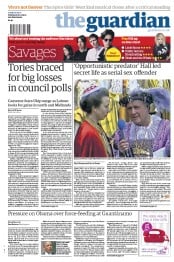A meticulously arranged shot on a white background features a central guardian figure skewed slightly to the left. Surrounding this central piece are four smaller figures, possibly representing protectors or "savages," alongside four prominent council poles. The scene includes an image of a man and a woman, embedded within another article. Additionally, there is a partially legible headline, starting with a 'P' and resembling "Pressure on Obama over face feeding," followed by the location "Gastonia." It seems some people doubt whether this place is actually in America. The composition is intricate and appears to be rich with cultural and political symbolism.